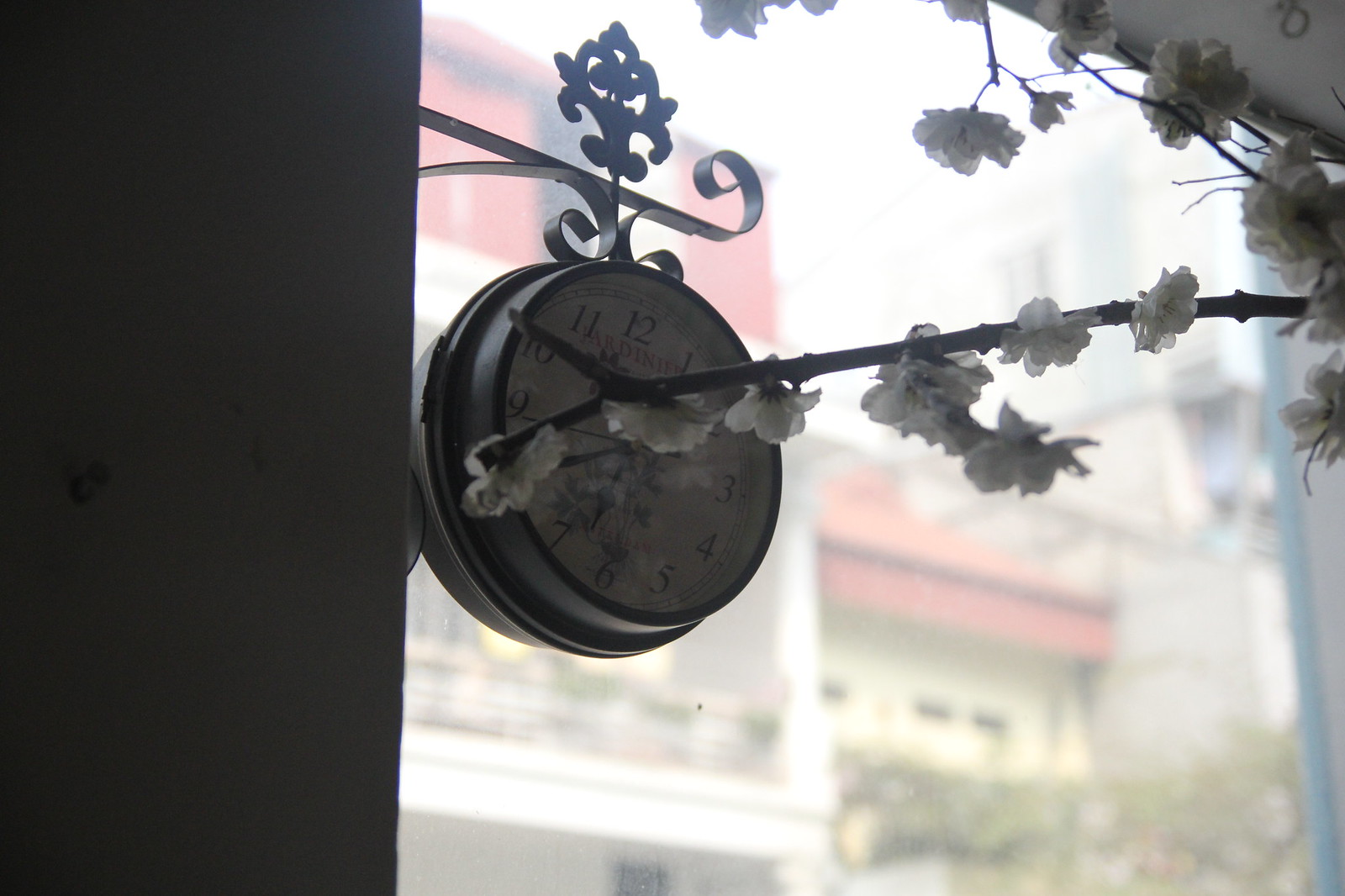The photo captures an intricate outdoor scene with a blend of natural and architectural elements. Central to the image is a round clock, adorned with conventional numbers from 1 to 12, hanging from an ornate black metal plant hanger affixed to a wall on the left side. The exact time on the clock remains hidden behind a delicate branch adorned with small white flowers. The background reveals the blurred, multi-leveled facade of a building, featuring red accents but largely rendered indistinct due to the bright lighting and focus. The perspective suggests the photo might be taken from within a store, looking through a window to the outside, with the clock seemingly suspended just outside. Ambient darkness inside contrasts starkly with the sunlit exterior, adding a layer of depth to the scene.